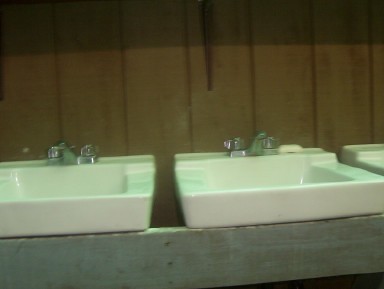This indoor photograph captures a pair of adjacent ceramic sinks, identical in their rectangular, deep design, seemingly brand-new with a sleek, polished white porcelain finish. Each sink is equipped with chrome faucets, featuring silver knobs presumably for temperature control. The sink on the left is slightly cut off by the image's edge, while the one on the right has an additional detail of a bar of soap resting on its surface. Below these sinks is a horizontal beam made to look like natural wood, but with a hint of gray, suggesting it's weathered or aged. A dark tan paneling, reminiscent of 1970s vinyl strips, forms the background. The image itself is slightly grainy, dark, and somewhat out of focus, with the upper portion particularly shadowed. The overall impression is of an outdated space, perhaps reminiscent of public restrooms found in malls, movie theaters, or parks.